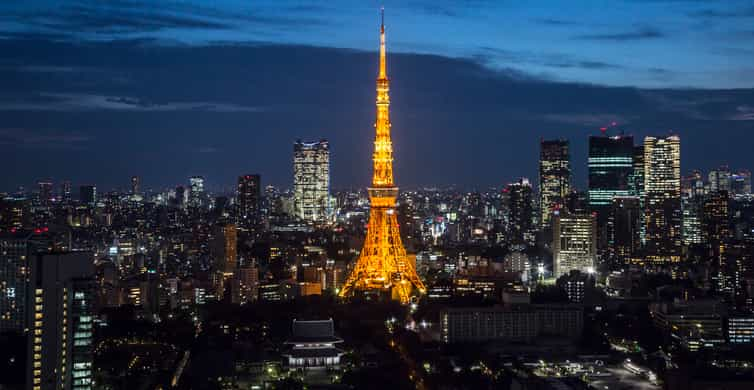The image captures a breathtaking nighttime view of the Paris skyline with the iconic Eiffel Tower illuminated in a rich orange-yellow hue, standing majestically in the center. The scene unfolds in a horizontally rectangular frame, showcasing a city bustling with lights as twilight wraps the horizon. The dark blue-gray sky hints at an impending sunset, creating a serene backdrop for the twinkling cityscape. Surrounding the Eiffel Tower are various buildings, their windows aglow, highlighting the vibrancy of the metropolis. The entire composition exudes a tranquil yet dynamic atmosphere, with clusters of illuminated structures harmoniously enhancing the tower's radiant presence.